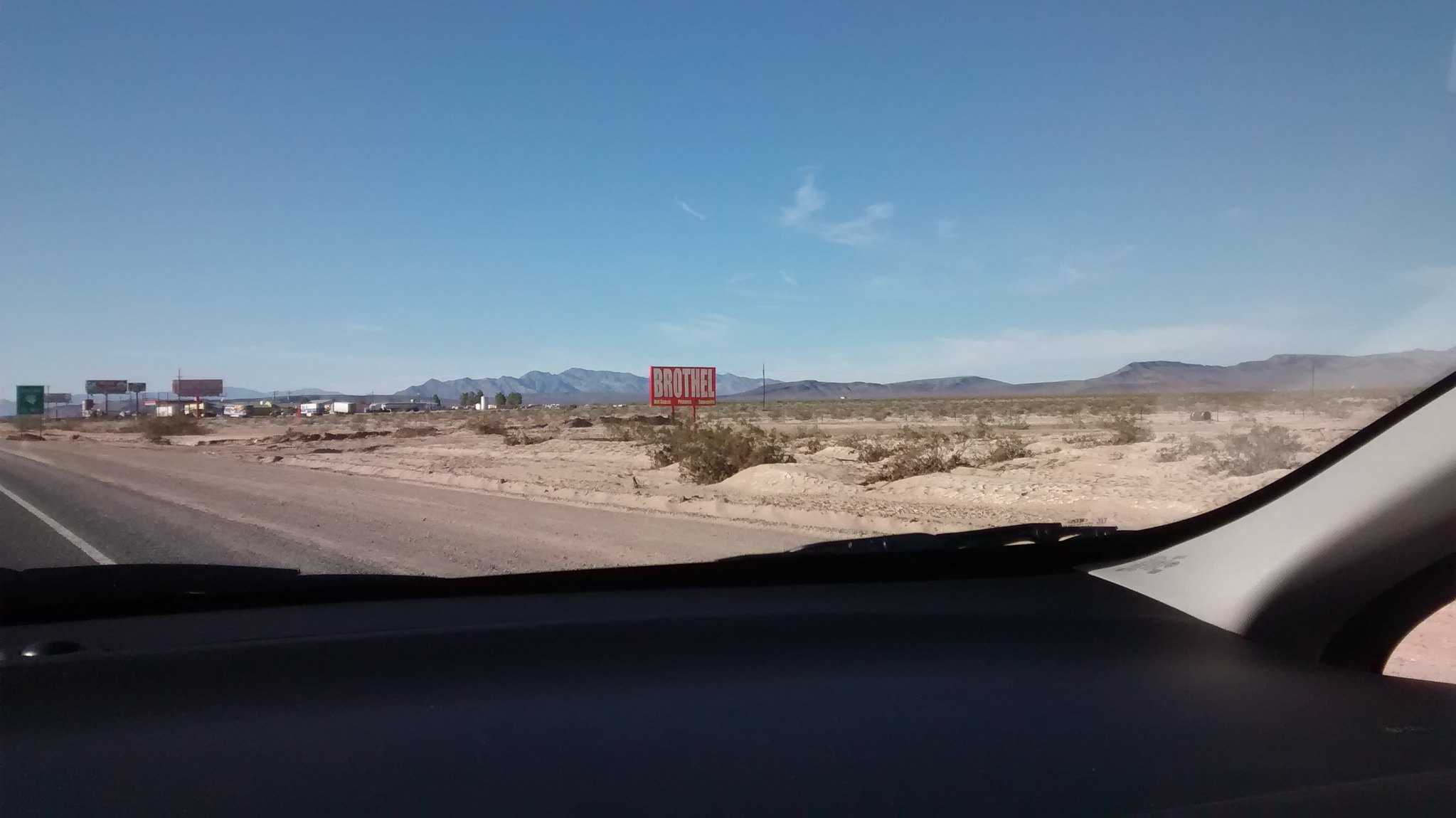This outdoor image, taken from the inside of a car, prominently features a dark dashboard. Beyond the windshield, a sprawling desert landscape unfolds under a vibrant blue sky scattered with fluffy white clouds. In the middle distance, a red building with the word "Brothel" written on it can be seen amidst a sea of shrubbery. Distant mountains loom in the background, providing a dramatic backdrop to the scene. Scattered buildings and billboards dot the far reaches of the horizon, while a black asphalt road cuts through the desolate beauty of the desert.